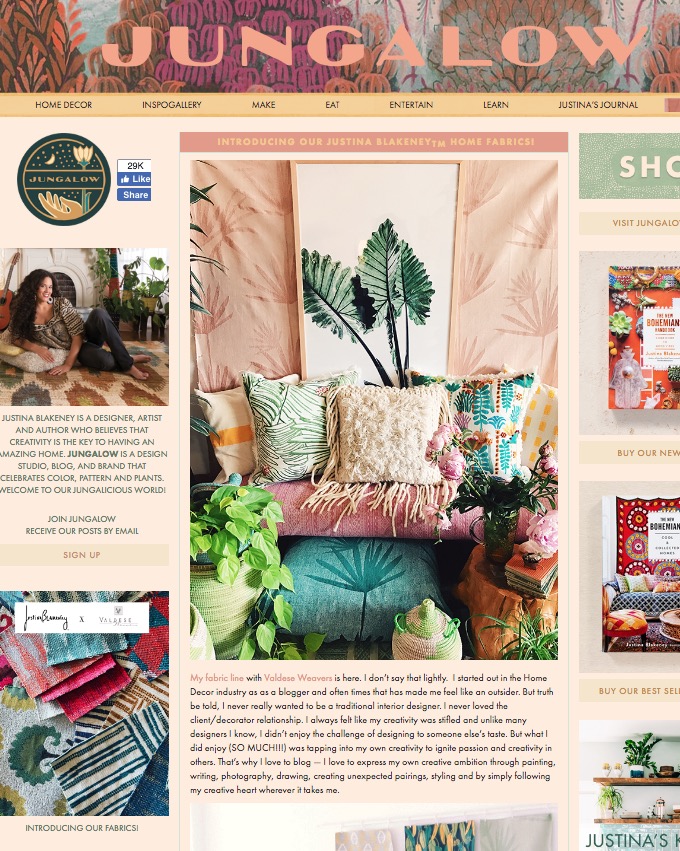This image appears to be a screenshot from a website or a magazine page, prominently titled "Jungalow" in pink with a flowery design at the top featuring pastel colors like pinks, purples, and oranges. Just below the title, there's a yellow navigation bar with sections including 'home decor', 'inspo gallery', 'make', 'eat', 'entertain', 'learn', and 'Justina's journal'. In the center of the page is a large photo showcasing a pink bench against a tapestry adorned with palm leaves. The bench is accessorized with a variety of colorful, fringed decorative pillows, a green fabricated stool, and other miscellaneous items. Surrounding the bench are numerous houseplants and additional greenery, enhancing the tropical and vibrant aesthetic. A framed picture of large green leaves and a peach-colored drape with leaf motifs hang behind the bench. To the right side, there are promotional texts about purchasing books, encouraging visitors to buy their new or best-selling titles. On the left, there is an image of Justina Blakeney, a designer, possibly the creator of the content, lying on a rug. The bottom section of the page features fabric swatches available for selection, indicating the theme of home decor and textiles. Additionally, there are social media links at the top left for Facebook, an article introduction in the center frame, and a call to sign up for a newsletter or shop for featured products on the right.